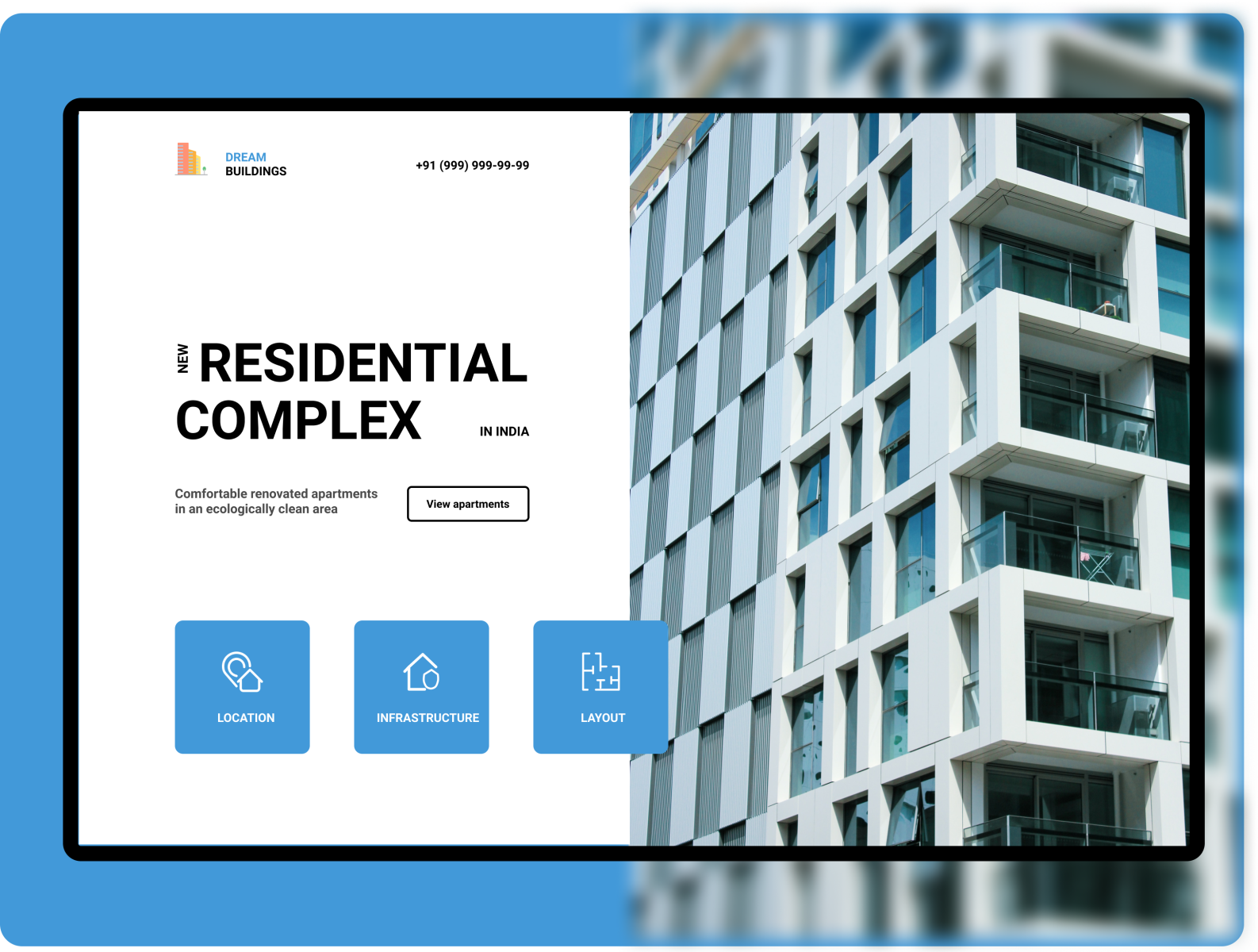**Advertisement for New Residential Complex in India**

The webpage features an advertisement for "Dream Buildings," showcasing a modern residential complex in India. Dominating the center is a high-resolution image of a pristine white apartment building with innovative architectural elements and multiple balconies. 

On the image, in large, bold text, it states "New Residential Complex in India," emphasizing comfortable, newly renovated apartments situated in an ecologically clean area. 

There are three blue squares beneath this, each containing white line-drawing icons:
- **Location**: Depicted by a house outline with a geotag icon, indicating ease of access and a desirable setting.
- **Infrastructure**: Illustrated by a house with a small garden, suggesting well-developed surroundings with essential amenities.
- **Layout**: Shown by a floor plan, hinting at thoughtful and practical apartment designs. 

These details are all enclosed within a prominent black box, making the information stand out against a blurred background. This blurred section surrounds the black box and seamlessly transitions into a serene, blue sky backdrop, which enhances the visual appeal of the advertisement.

Additionally, the advertisement provides a contact number: +91 999 999 9999, indicating the potential for inquiries or further details.